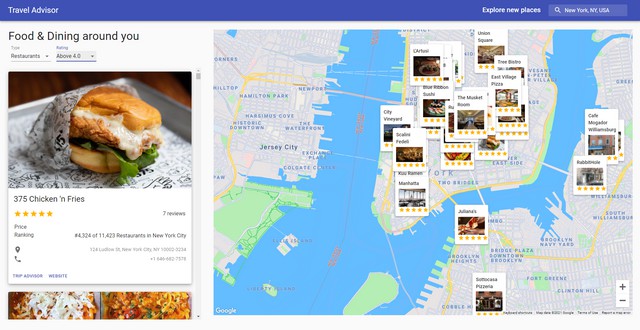The screen capture showcases a detailed and dynamic travel advisor page focused on food and dining options. The page includes a search for restaurants near your location that boast ratings of 4.0 and above. Featured prominently is an image of a popular dish titled "375 Chicken and Fries," displaying a tempting tray lined with white greaseproof paper. The tray holds a sandwich with a fried chicken patty, melted cheese, and fresh lettuce nestled in a bun.

This restaurant has garnered 7 reviews and falls within the price range of over $4,224 out of $11,473, highlighting its premium standing in New York City's dining scene. The restaurant's address appears to be around 728 Ludlum, though the image resolution makes it difficult to confirm the exact location.

Beneath this main image is a thumbnail showcasing side-by-side pictures of what appears to be bruschetta or similar elegantly presented dishes, suggesting a variety of culinary options.

Dominating the main section of the screen is a comprehensive map of Manhattan, New York City. This map extends to also display parts of Jersey City, Brooklyn Heights, and South Williamsburg. Although there are various restaurant pop-ups in Manhattan and Brooklyn Heights, Jersey City is devoid of any restaurant icons. The map designates the cities in grey, the water bodies in pale blue, and park areas in green, facilitating easy navigation. The page header invites users to "Explore New Places" in New York, New York, USA, encouraging culinary adventures across the city.